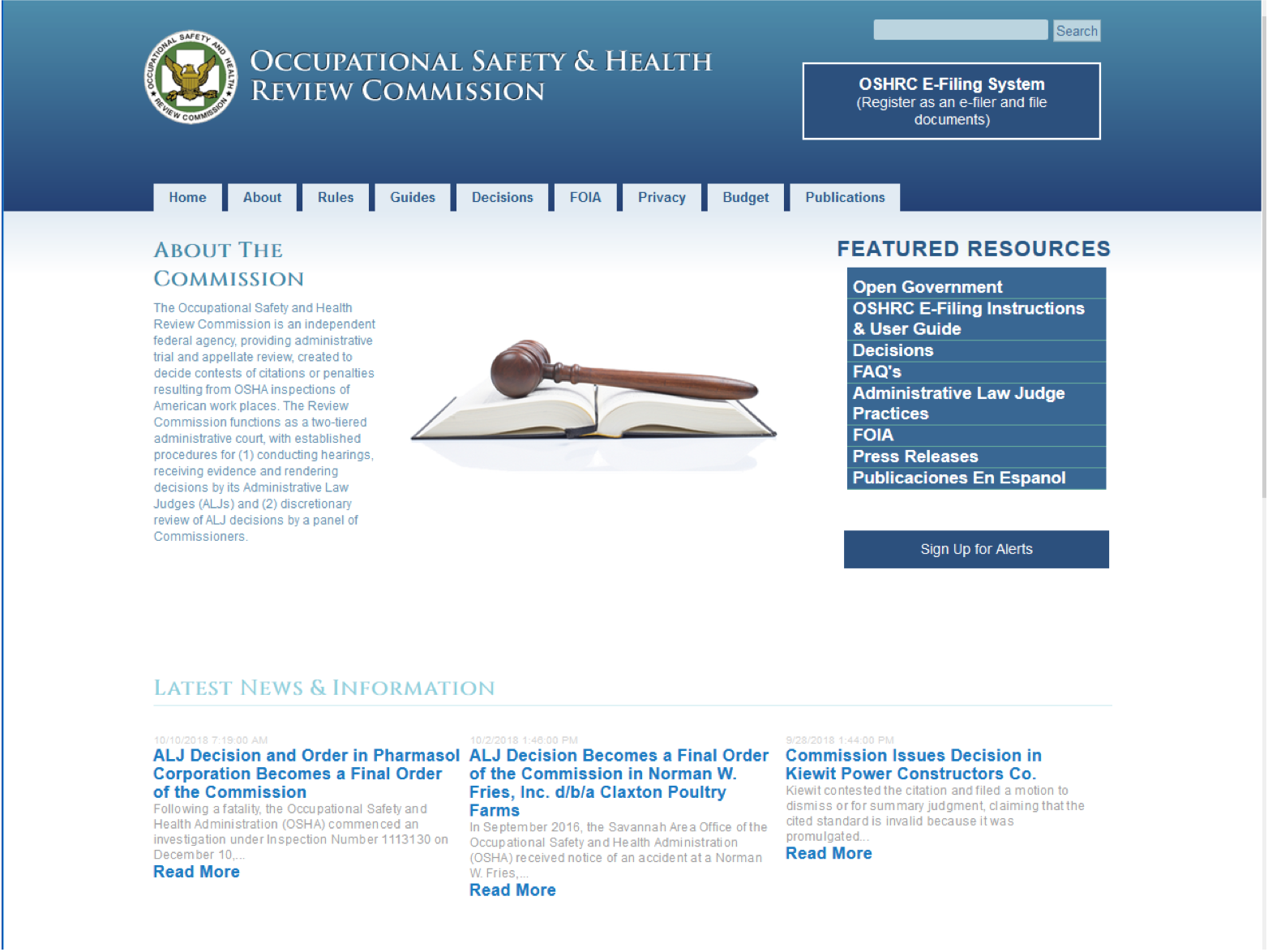Here is a detailed and cleaned-up version of the descriptive caption:

"The webpage features a primarily white background with a prominent blue header. At the top, the title 'Occupational Safety and Health Review Commission' is displayed alongside a logo on the left, depicting an eagle with a white cross behind it. To the right of the logo, there is text that reads 'OSHRC e-filing system: Register as an e-filer and file documents.' Below the header, a navigation bar includes various tabs: Home, About, Rules, Guides, Decisions, FOIA, Privacy, Budget, and Publications.

Scrolling down, there is a section titled 'About the Commission.' This part elaborates that the Occupational Safety and Health Review Commission is an independent federal agency tasked with providing administrative trial and appellate review. It was established to resolve contests of citations and penalties stemming from OSHA inspections of American workplaces. The Review Commission operates as a two-tiered administrative court. The first tier involves conducting hearings, receiving evidence, and rendering decisions by its Administrative Law Judges (ALJs). The second tier involves discretionary review of ALJ decisions by a panel of commissioners.

At the bottom of the page, there are clickable links titled 'Latest News' and 'Information,' providing users with quick access to the most recent updates and relevant data."